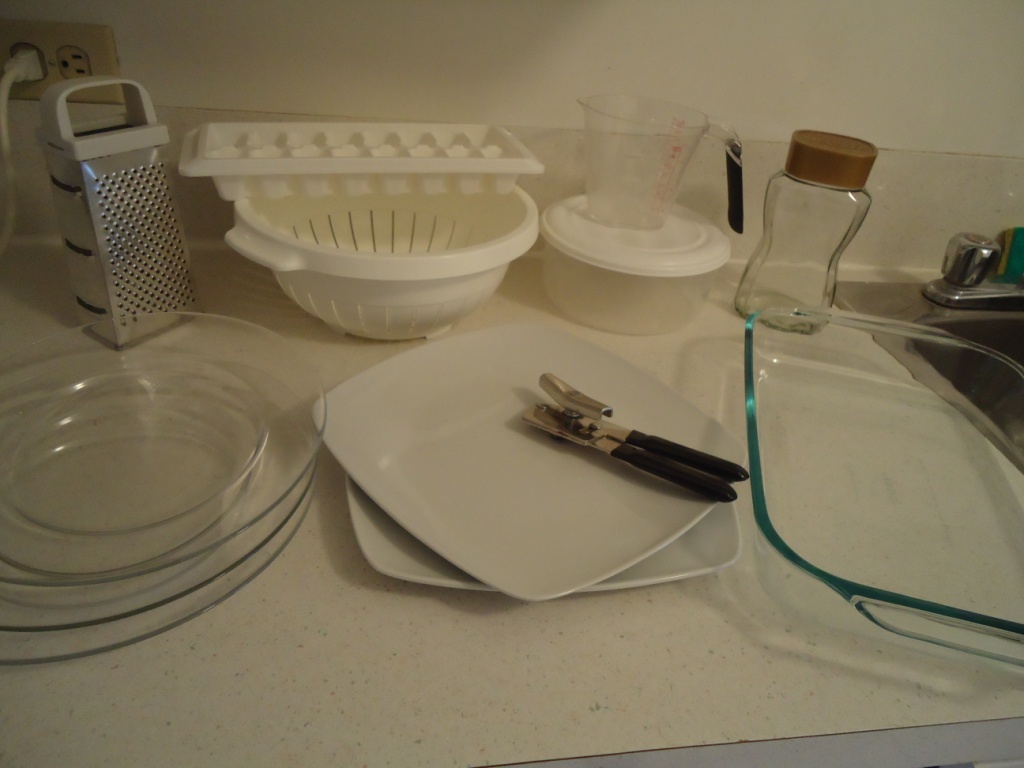This vibrant and detailed color photograph captures the interior of a cozy home, focusing on a well-used kitchen countertop. To the right, a partial view of a stainless steel sink is visible, showcasing one of its gleaming faucets. Centered prominently on the counter is a clear glass baking dish, ready for use in the oven. Situated just behind the baking dish is a clear jar with a distinctive brown lid.

To the left of the scene, a variety of kitchen items are meticulously arranged. A clear measuring cup and a piece of Tupperware with a white lid sit alongside a stack of pristine white plates. On top of the topmost plate rests a black-handled can opener. Adjacent to these items, a set of three clear glass plates are neatly stacked, with a bowl perched on top. Further back, a white colander and an ice tray lean against the backdrop, contributing to the organized clutter. Completing the kitchen ensemble, a metal grater stands ready for use nearby.

Additionally, the photograph features a detail of a wall socket, with a single white cord plugged in, emphasizing the everyday functionality of this homey kitchen space.